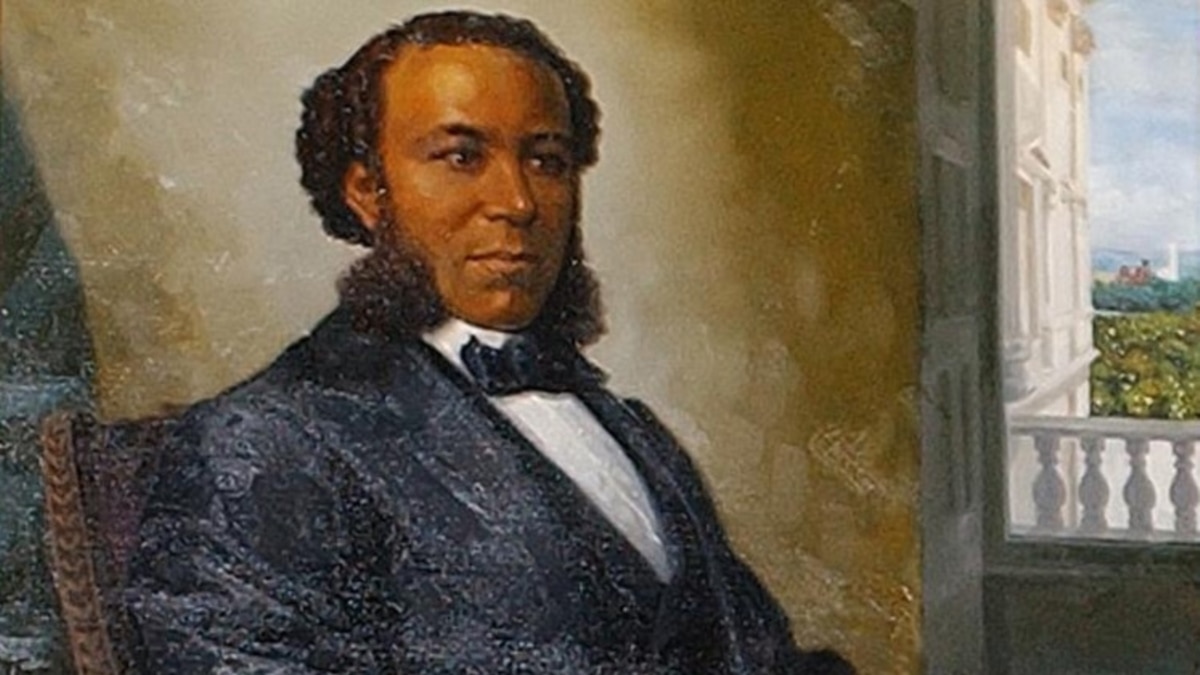The image is a detailed painting of a young Black man, exuding a sense of prestige reminiscent of the mid to late 1800s. He is seated in an intricately designed chair featuring a series of V-shaped patterns along its side, posed next to an open window that leads to a balcony with white railings and a colonnade. The backdrop of the painting includes a light tan wall and a view of a blue sky with distant mountains, which enhances the serene atmosphere.

The man has well-groomed, short, curly black hair and curly black sideburns that extend down to his jawline, resembling the prominent sideburns of Elvis Presley in their fluffy and voluminous nature. His expression is semi-stoic as he gazes off to the right. He is dressed in a distinguished black jacket, a black bow tie, and a crisp white shirt, highlighting his gentlemanly and affluent appearance. The overall composition suggests a setting within a prestigious household, reinforcing the man's status and elegance.